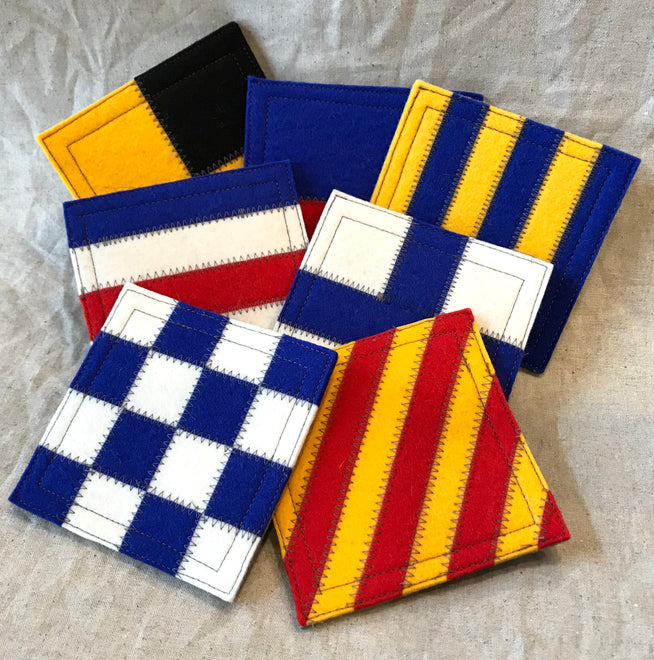The photograph features an arrangement of seven handmade square coasters with various patterns, laid out on a heavily wrinkled gray fabric with sporadic gray dots. The coasters, stitched together from different felt panels, have a distinct nautical theme. The foremost coaster in the array is a blue and white checkerboard pattern. Behind it, there’s a yellow and blue striped square, and next to it, a white square with a prominent blue cross. Continuing back, there’s a square with blue stripes at the top, white and red stripes in alternating sequence. Beneath that, a square divided into half blue (top) and half red (bottom) can be seen. The backmost coaster has a top left and bottom right corner in yellow, with a black top right corner, although part of it is obscured by the other coasters. All the coasters have visible stitching along the edges, highlighting their handmade quality.